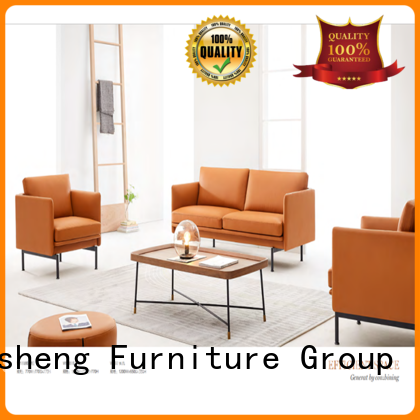The image depicts a staged living room setting designed to showcase various pieces of furniture, all enclosed by a solid orange frame. Central to the image is a coffee table placed atop a rug, surrounded by a loveseat to the top-right, single chairs to the left and right—with one chair partially out of the frame—and an ottoman positioned below and to the left of the table. In the background, there is a ladder that might be a towel rack or mirror, and a wall with some hanging items. The floor is white with a centrally located carpet.

Prominently displayed text includes “100% Quality, Quality 100% Guaranteed,” along with “Sheng Furniture Group” placed at both the top and bottom of the image in black letters. The image's colors are a blend of orange, white, tan, gray, green, gold, and black, creating a cohesive yet diverse palette. The furniture pieces and the other objects are scattered around the space, giving it an intentional, artfully disordered appearance. The overall setting is likely an advertisement for a furniture store, emphasizing the quality and variety of the products on display.